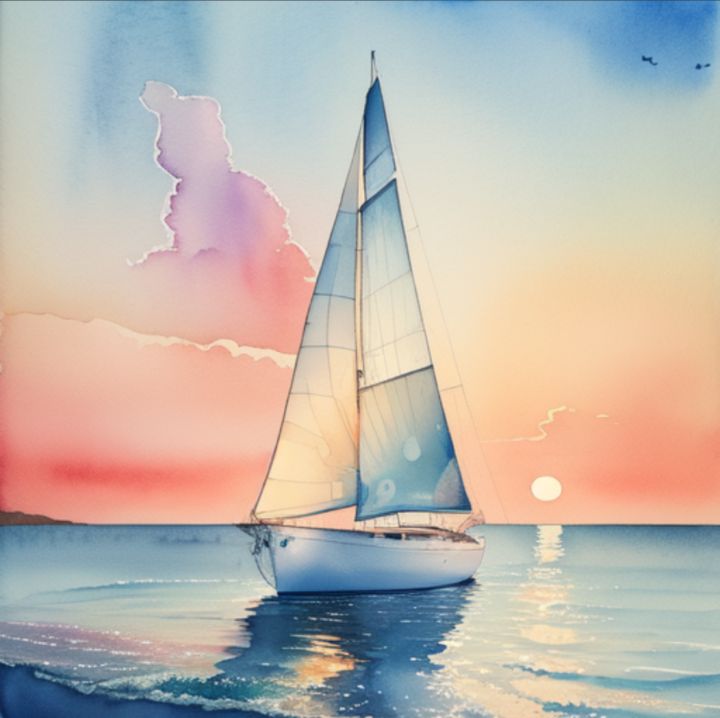This image, which appears to be either a watercolor, digital, or oil-based painting, depicts a serene maritime scene with great detail. The large, centrally positioned sailboat has tall, thin sails in shades of beige and blue. The boat itself is white and appears to be unoccupied. The water beneath it is a bluish-gray hue, gently rippled with little white caps. In the lower left corner, the dark gray shoreline just peeks into view.

Above, the sky is an exquisite gradient, transitioning from coral and pink hues around a setting sun—a perfect yellow circle situated just behind the boat to the right—into shades of white and blue, with the upper right corner being particularly vibrant. To the left of the sail, a cloud showcases a mix of purple and pink. Additionally, two small black v-shaped birds can be seen soaring in the upper right section of the sky. This expertly crafted artwork beautifully captures the tranquil essence of a sailboat at sunset, set against a multicolored sky and gently rippling waters.